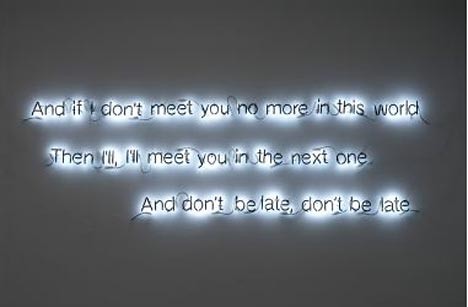The image features a rectangular black box, approximately 4 to 5 inches wide and 3 to 4 inches tall, set against a gray backdrop. Within the box, there are words inscribed in black text, made slightly more legible by a white, blurry highlight. The text reads: "And if I don't meet you no more in this world, then I will meet you in the next one. And don't be late, don't be late." The overall aesthetic is eerie and haunting, reminiscent of a message from the afterlife or a ghostly whisper. The message seems to imply a promise of reunion in the next life, urging punctuality in a somewhat unsettling manner. This text may be lyrics from a song, imbuing the image with an emotional and spiritual undertone.